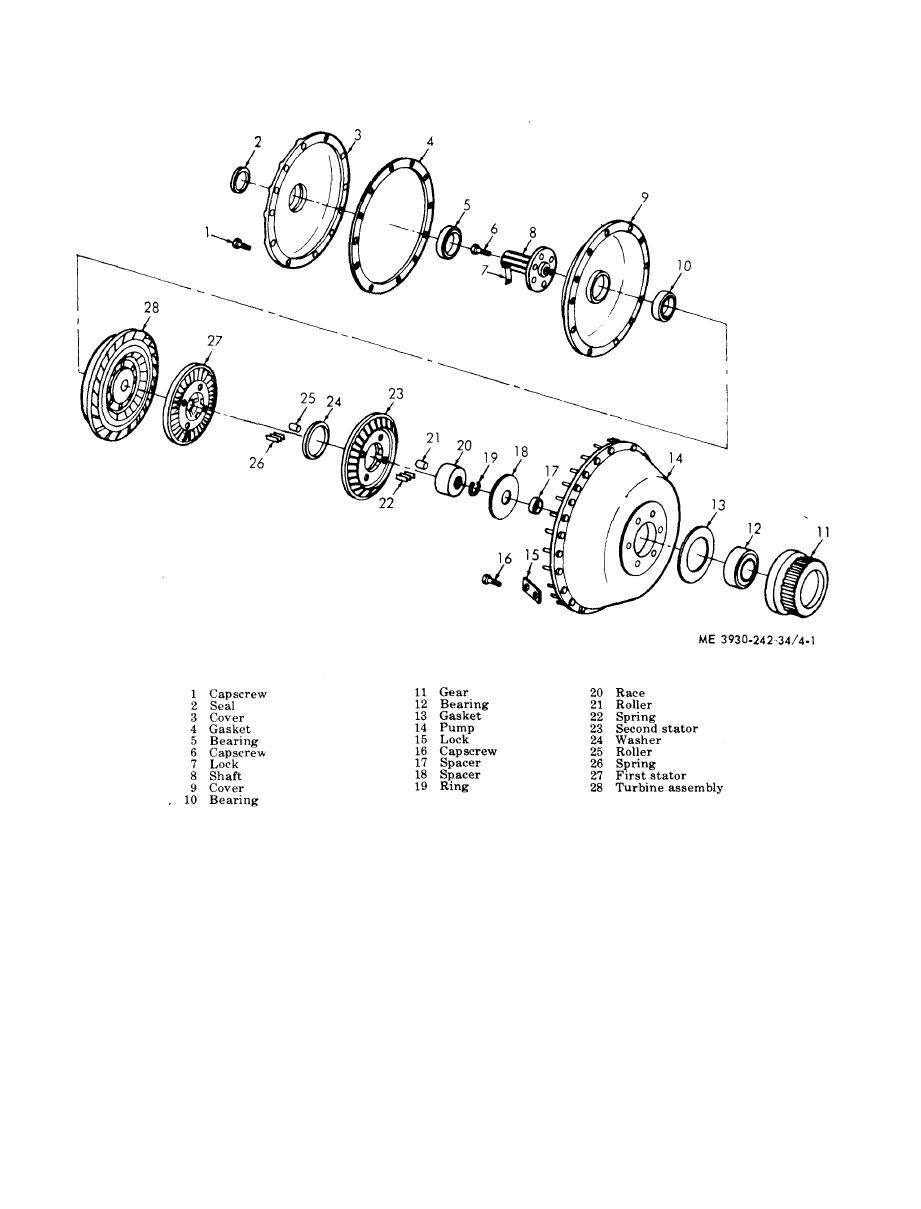The image is a detailed black-and-white diagram on a white background, illustrating an assembly of various gears and circular components, possibly a torque converter. The components are organized in two diagonal rows. The top row includes numbers 1 to 10, starting with a cap screw labeled #1, followed by a small circle labeled #2, a larger circle with a hole in the center labeled #3, and continuing with items numbered up to 10. The bottom row begins from the right side with number 11 and continues to 28. Each component is carefully numbered, and lines run through their centers, indicating that the pieces are meant to be connected or joined together.

The diagram includes detailed labels for each numbered part, forming three columns of text at the bottom. These labels provide the names of the components, such as cap screw, seal, cover, gasket, bearing, lock, shaft, gear, pump, spacer, ring, race, roller, spring, stators, and turbine assembly. The components are described as follows: 
1. Cap screw
2. Seal
3. Cover
4. Gasket
5. Bearing
6. Cap screw
7. Lock
8. Shaft 
9. Cover
10. Bearing
11. Gear
12. Bearing 
13. Gasket 
14. Pump
15. Lock
16. Cap screw
17. Spacer 
18. Spacer
19. Ring
20. Race
21. Roller
22. Spring
23. Second stator
24. Washer
25. Roller
26. Spring
27. First stator
28. Turbine assembly

Additionally, the annotation "ME3930-242-34-4-1" can be seen on the bottom right of the diagram.